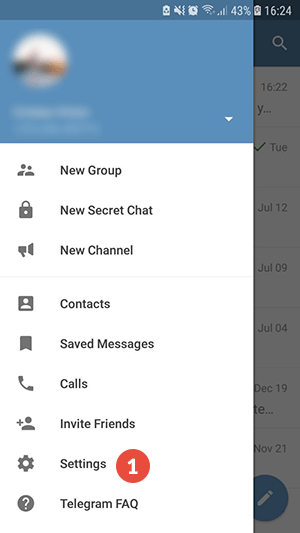This is a detailed caption for the image described:

"A screenshot from a mobile phone displays a translucent status bar at the top, showing the time as 16:24, a battery level of 43%, and icons for Wi-Fi, audio, and an alarm clock. Below the status bar, a purple square appears censored. Further down, there is a vertical list with options in dark gray font. The first item, 'New Group,' is accompanied by an icon of two human silhouettes. Underneath, 'New Secret Chat' is displayed next to a lock icon. Following that, a megaphone icon precedes the 'New Channel' option. Next, 'Contacts' is listed alongside an icon of a square containing a human silhouette. Below this, a bookmark icon is paired with the label 'Saved Messages.' The 'Calls' option, featuring a phone handset icon, is listed next, followed by 'Invite Friends,' represented by a human silhouette with a plus sign. At the bottom of the list, an icon of a gear is labeled 'Settings,' with a red circle containing a white '1' next to it."